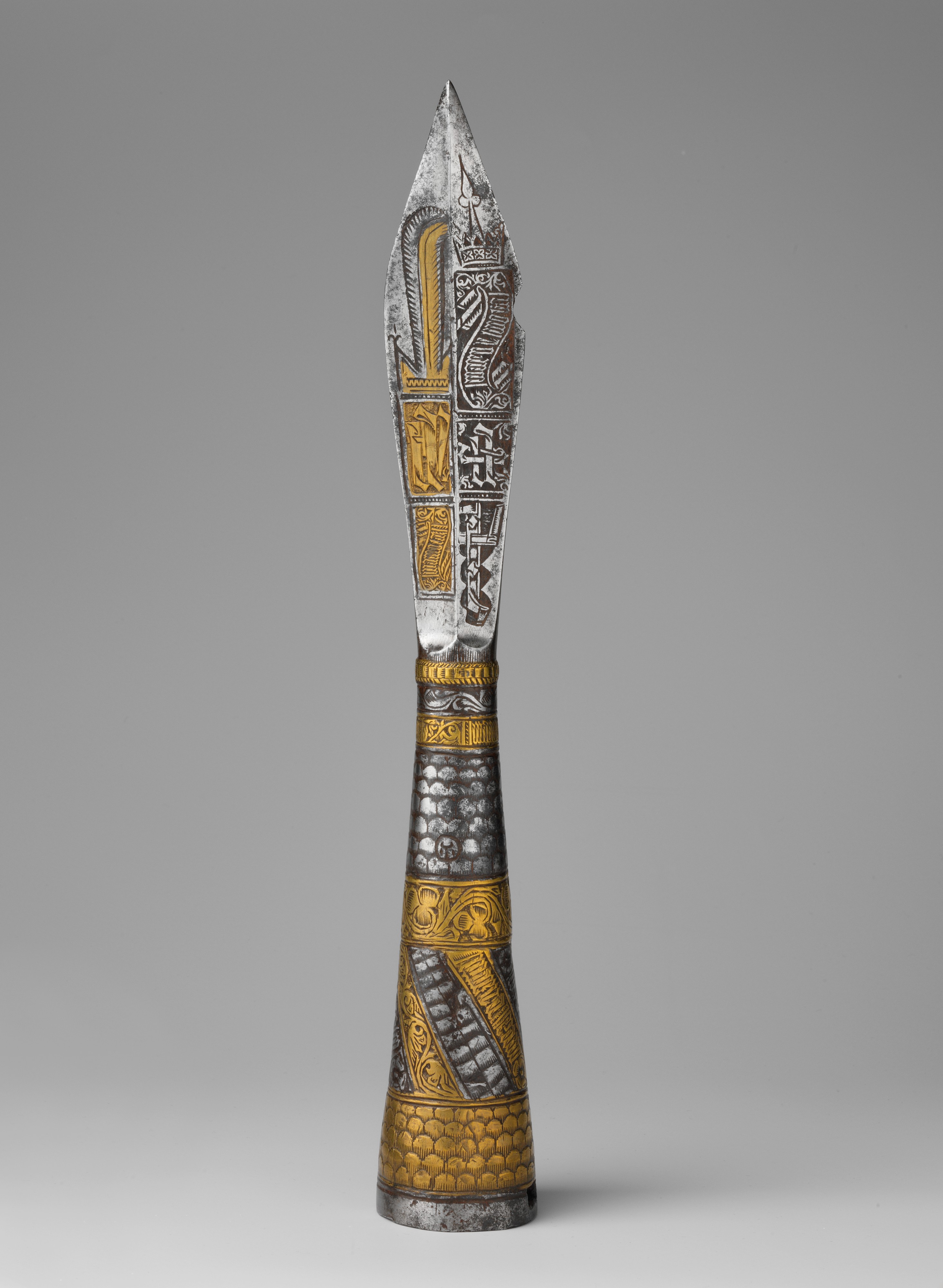The image depicts a highly detailed, color photograph of an antique ceremonial spearhead, presented against a flat, dark gray backdrop that creates the effect of it floating in an empty gray void. The spearhead is beautifully crafted, consisting of a tall, cylindrical shape that flares out slightly near the top point and the base, and narrows around the midsection. The upper section of the spearhead features a triangular, leaf-shaped tip made of steel, supported by a pewter-colored segment. Below the tip, the spearhead showcases an array of exquisite etched and engraved designs in gold, silver, black, and brass colors, with chrome accents. These intricate designs include circular patterns, scales, bricks, floral motifs, and a scroll, artfully arranged to create an overall cohesive and ornamental pattern. This elaborate craftsmanship along with its archaic form suggests its historical significance as an artifact and possibly a ritualistic or ceremonial item.